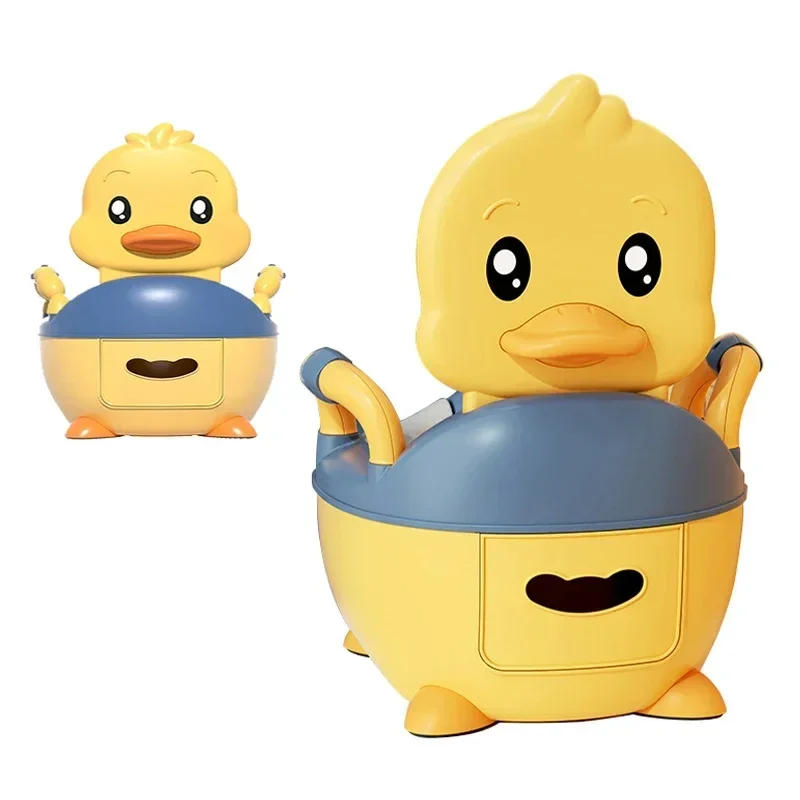The image features two views of a child's toy that resembles a yellow duck, which might function as a potty training chair. The toy has a large, plasticky duck face with a wide yellow beak, oval black eyes with white pupils, and subtle eyebrows. Notably, the ducks have slightly different hairstyles, with one sporting three tufts of hair and the other two.

Each duck has blue overalls, and what looks like handles on the sides could represent its arms. They stand on four yellow feet. The ducks feature a blue midsection, which might act as a lid or seat cover, leading to speculation that the toy may have a storage or functional use. Each duck has a slot in the belly area, suggesting that items could be stored inside or it might be part of its potty training functionality.

The background is white, accentuating the details of the ducks. One duck is presented closer to the viewer, positioned on the right side of the image, while the other is seen from a distance in the upper left corner, both displayed from slightly different angles to showcase more details. The toy’s basic pastel colors and cheerful appearance clearly aim at young children, likely to engage them in potty training activities.